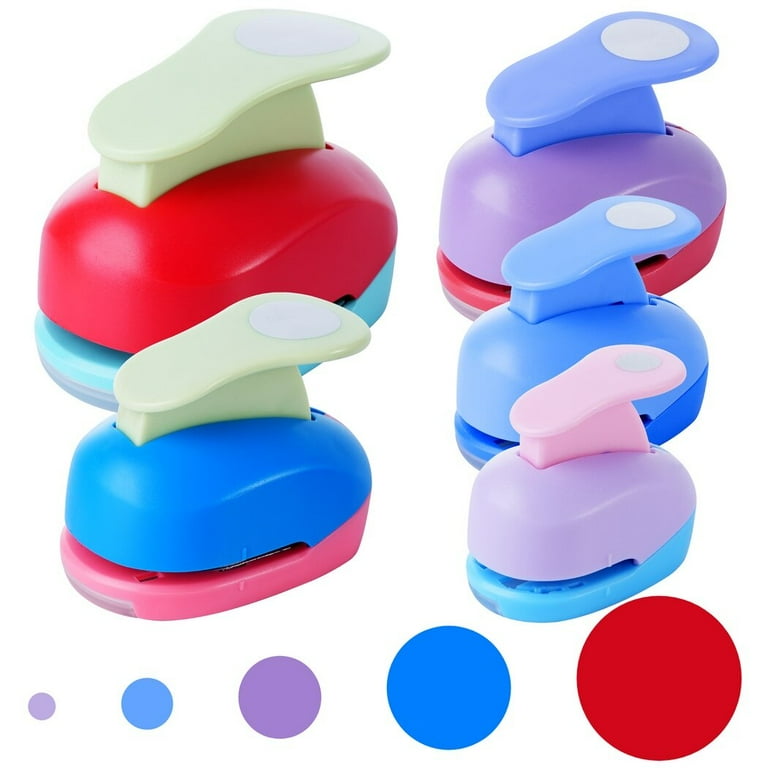The image features five colorful, toy-like objects that resemble small plastic staplers or stamps, and they are arranged against a white background. On the left, the front object has a rounded blue head with a white tab for pressing, and a pink base. Behind it is a slightly larger one with a red dome top, a light blue base, and the same white tab. On the right side are three more in varying sizes. The first has a purple and red theme with a blue tab, the second is blue with a darker blue base and a blue tab, and the last one combines purple and blue with a pink tab. All these objects have a slot where paper could be inserted, and a lever on top for pressing down, hinting at their function as either staplers or stamps. Below these objects are five circles of different sizes and colors: a tiny purple circle, a blue circle, a darker purple circle, a darker blue circle, and a large red circle, from left to right. The arrangement and the white background suggest that this might be an advertisement display.